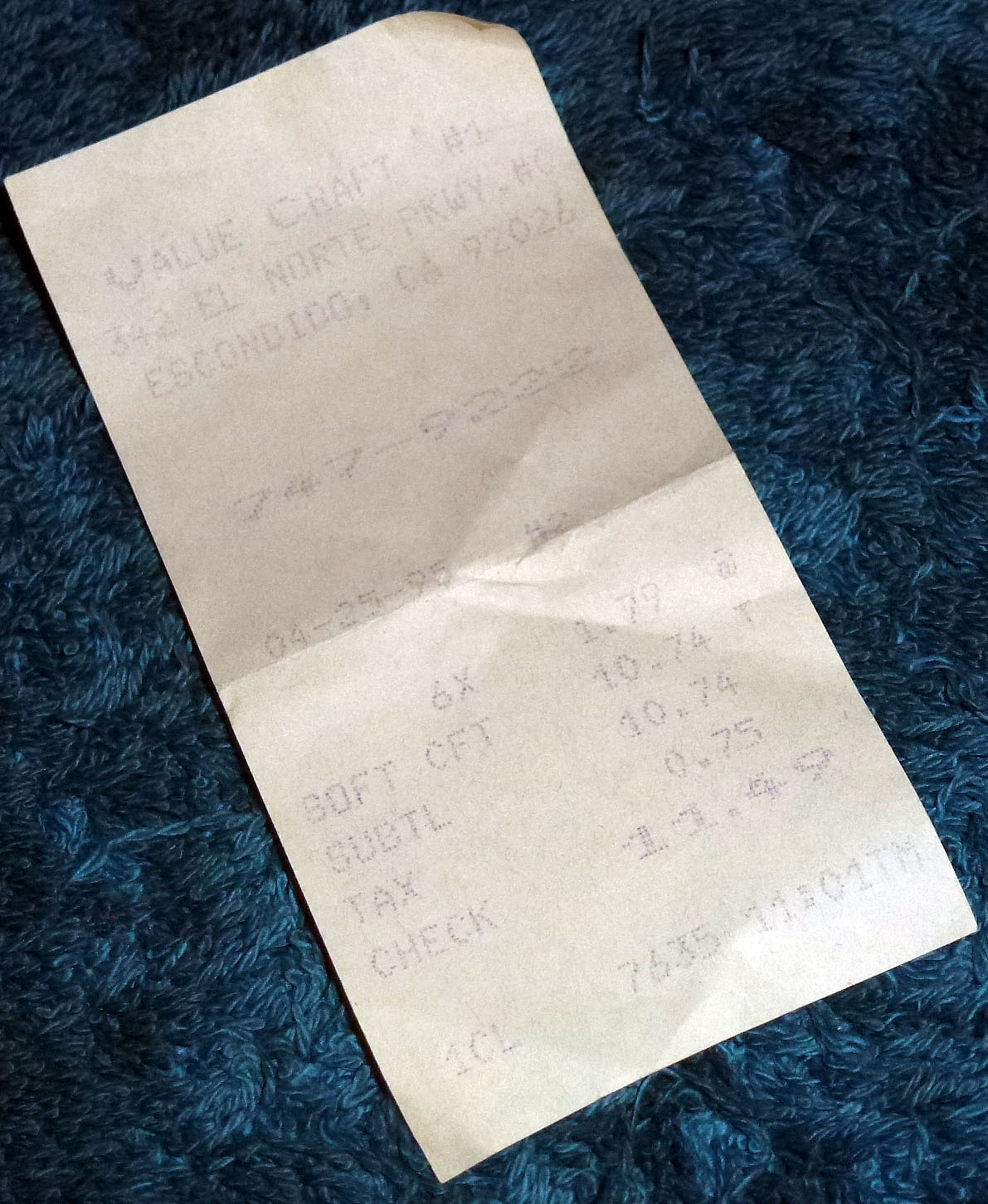In the photograph, an old, faded receipt from ValueCraft rests on a retro-style blue shag carpet, reminiscent of the 1980s with its long, furry strands. The receipt paper appears coarse and rough, unlike modern receipts. The text, although faded, indicates the address as 342 El Norte Parkway, Escondido, California, 92026, with the phone number 747-9223. Dated April 25th, 1995, the nearly 30-year-old receipt details a purchase of "soft CFT" for $10.74, with an additional tax of 75 cents, bringing the total to $11.49. The transaction was recorded at 11:01, though it is unclear if it was AM or PM. The receipt, folded and showing signs of age, captures a snapshot of daily life from the mid-90s.